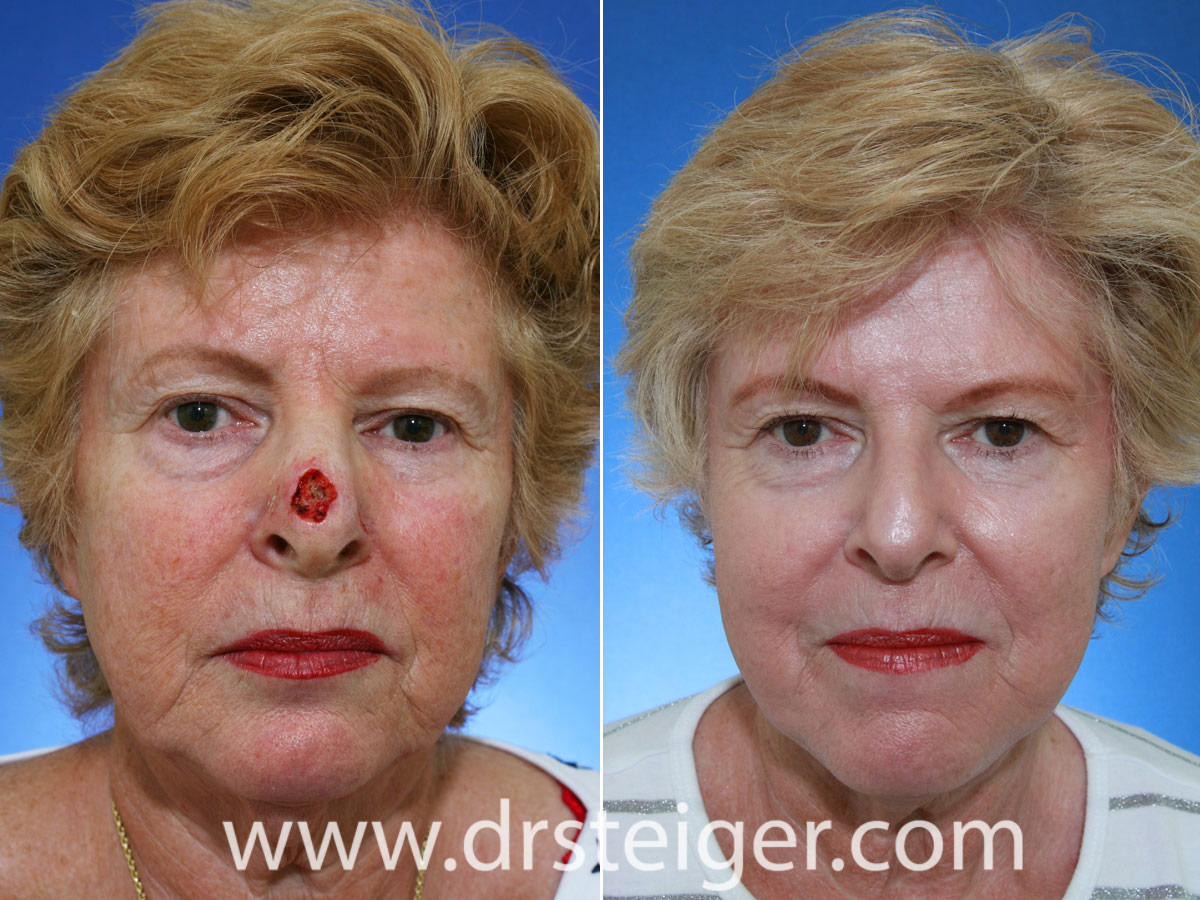The image features two side-by-side photographs of the same older woman, seemingly in her 60s, set against a blue background. Both images display the URL www.drstiger.com at the bottom. In the photograph on the left, the woman has short, curly brown hair, dark irises, and is wearing red lipstick. She is dressed in a shirt that exposes her neck, adorned with a gold necklace. Notably, she has a large, gruesome lesion on her nose, described as blood-red with black splotches, and her skin appears darker and more sun-damaged. 

In contrast, the right photograph shows the same woman with lighter, reddish-blonde hair, a slightly paler complexion, and thinner eyebrows. The wound on her nose is completely healed, leaving her skin with a more even pinkish tone. She is also wearing red lipstick and a white top with gray stripes. Both images capture her looking directly at the camera. The transformations in her appearance suggest she may have undergone cosmetic or medical treatment.